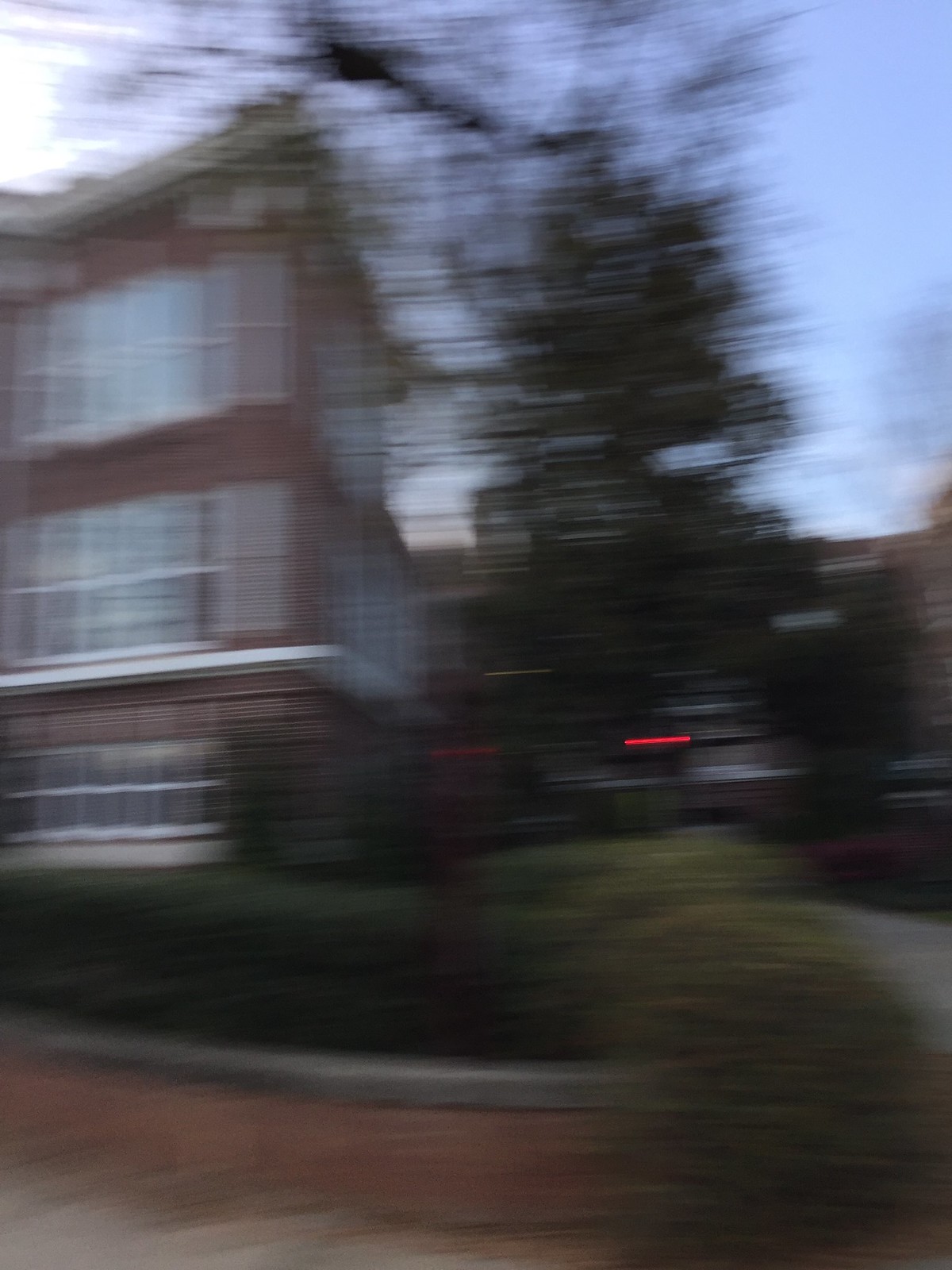This photograph, presented in a vertical rectangular format, showcases a partially visible three-storied brick building on the left-hand side. The structure is characterized by large windows on each story that hint at its residential or institutional nature. The red brick facade is complemented by concrete trim near the top and white trim around the first floor. 

In the bottom right corner of the building, a bush and a patch of grass are visible, leading down to a curb. Below the curb is a red brick road that adds texture and color to the scene. To the right of the building, a large evergreen tree with red lights beneath it suggests the presence of a deck or outdoor living space. The background is framed by a vivid blue sky, enhancing the overall atmosphere of the image. Despite the blurriness, the photo captures the quaint charm and architectural details of the setting.